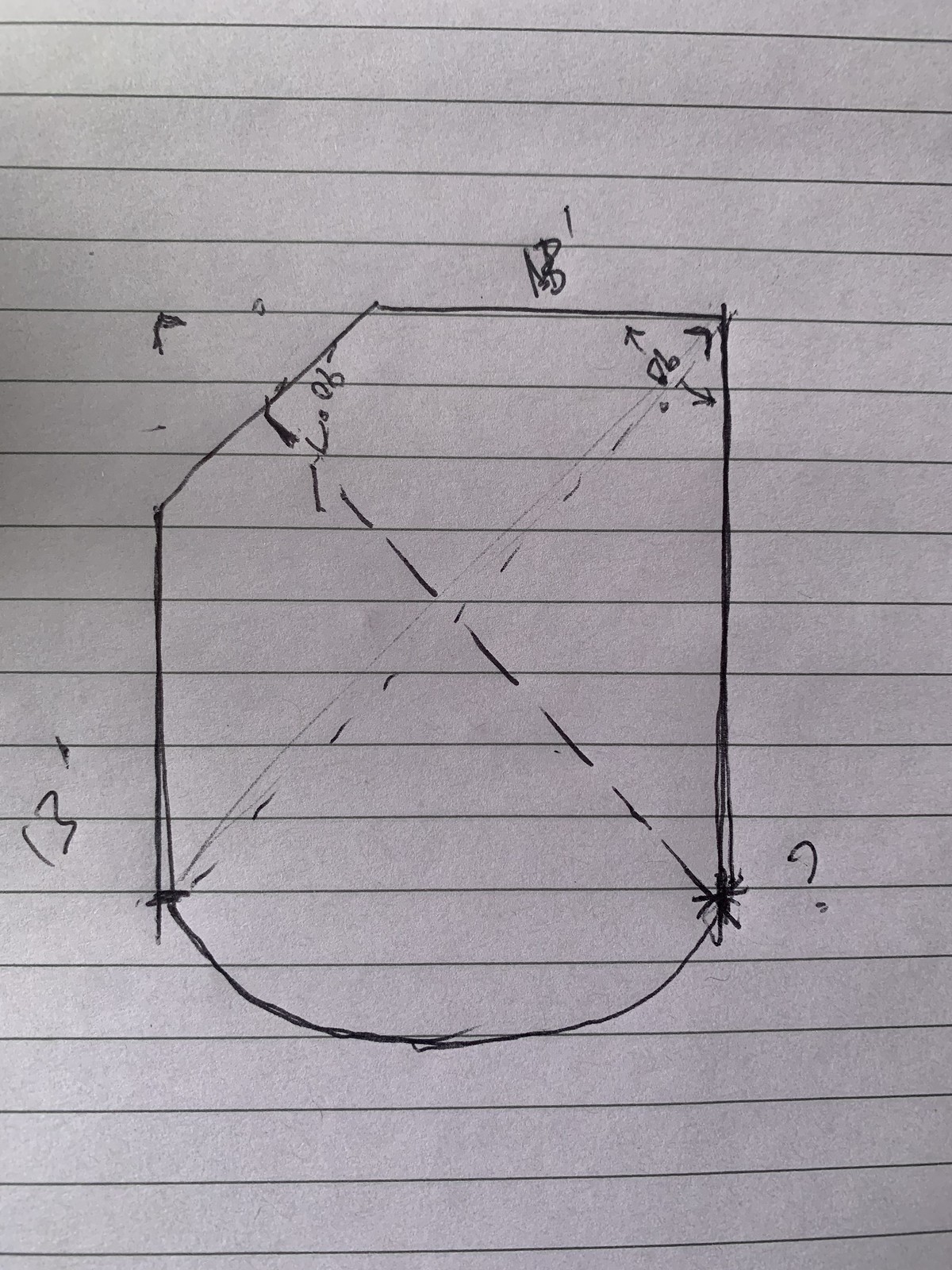This image features a meticulously hand-drawn sketch on white, lined notebook paper. The focal point of the drawing is an oddly shaped structure, beginning with a curved bottom edge that seamlessly transitions into a rectangular form. Intriguingly, a diamond-shaped section appears to have been cut out from this rectangle. The overall design suggests an architectural or construction blueprint.

Central to the drawing are carefully placed diagonal dashes that span across the middle, perhaps indicating a pattern or measurement detail. There are multiple numerical notations surrounding the structure, which seem to represent various dimensions or measurements, although some are not entirely legible.

Notable annotations include a measurement denoted as either '06' or '90', depicted with arrows pointing in opposite directions along one of the diagonal lines. Another diagonal line features a partially illegible notation followed by '06'. Measurements also appear along the sides of the rectangle: the shorter side is marked with '13', while the longer side is ambiguously labeled with just a question mark.

All elements of the sketch, including the measurements and dashed lines, are rendered in black ink. The entire drawing is oriented in portrait mode against the backdrop of white notebook paper with gray horizontal lines.